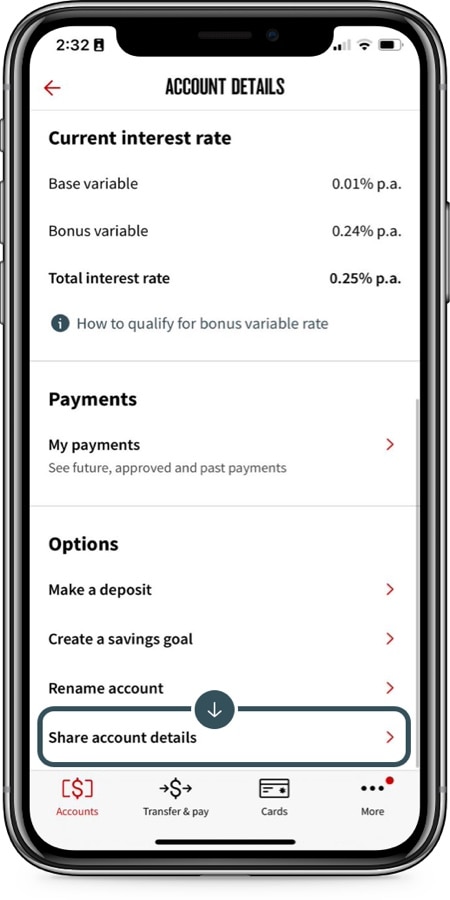A close-up image of a smartphone screen displaying a banking application. The time shown on the phone is 2:32. The device has two bars of cellular service and two bars of Wi-Fi connectivity, with the battery level at three-fourths full. The main screen features account details, including a breakdown of the current interest rates: a base variable rate of 0.01% PA, a bonus variable rate of 0.24% PA, and a total interest rate of 0.25% PA. Options to qualify for the bonus variable rate are also visible.

Below the interest rate details, there are various account management options such as "Payments," "My Payments," with sections for future, approved, and past payments. Additional options include "Make a Deposit," "Create a Savings Goal," "Rename Account," and "Share Account Details." 

The interface includes tabs labeled "Accounts" in red, "Transfer and Pay" with a cash symbol and arrows, "Cards," and "More," with a red dot indicator next to "More." The overall text is in black, set against a white background. The smartphone has a black border with three buttons on the left side and one button on the right side.